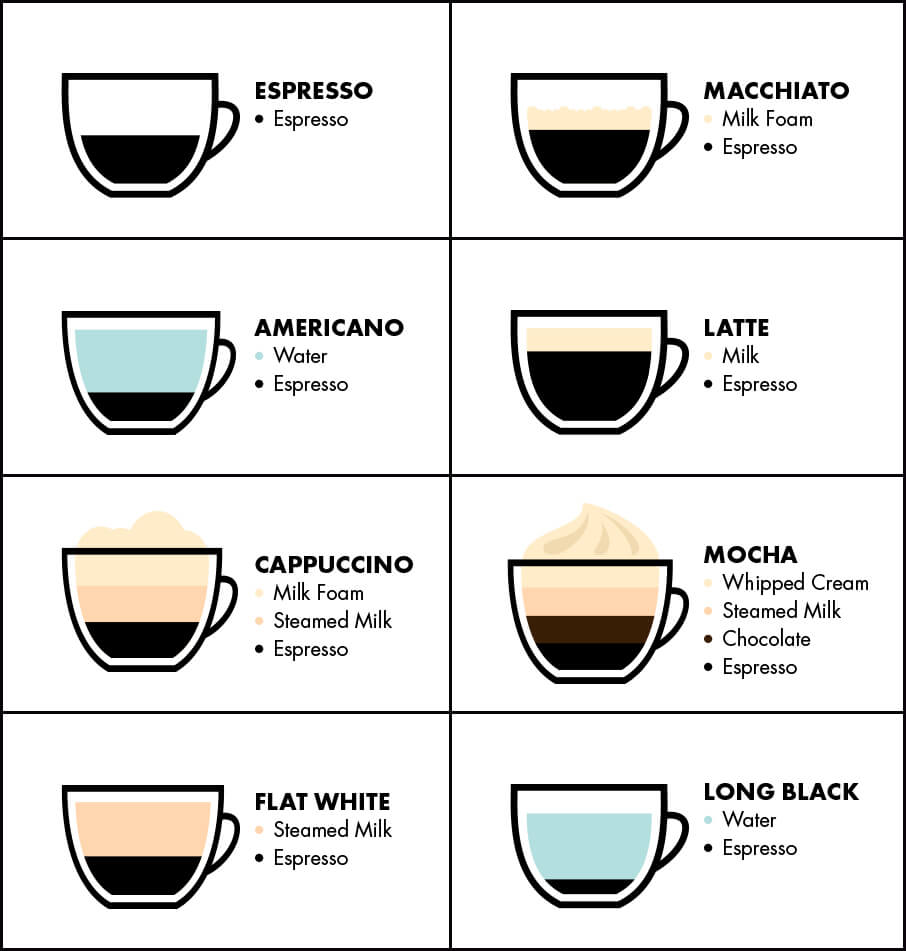This image, presented in portrait mode, is a detailed chart of different types of coffee, divided into eight segments. Each segment features an outlined coffee cup, illustrating the varying compositions and colors of each coffee type.

- **Top Left:** An espresso, depicted as a full cup of black coffee.
- **Top Right:** A macchiato, comprising a half cup of black coffee topped with an off-white milk foam.
- **Second Row Left:** An Americano, showing a small amount of black coffee with water filling the majority of the cup.
- **Second Row Right:** A latte, consisting of espresso with a significant portion of milk and a small layer of foam.
- **Third Row Left:** A cappuccino, with layers of espresso, steamed milk, and milk foam.
- **Third Row Right:** A mocha, featuring espresso, chocolate, steamed milk, and whipped cream on top.
- **Bottom Left:** A flat white, made up of espresso and steamed milk.
- **Bottom Right:** A long black, characterized by a small amount of espresso and a large amount of water.

The chart visually distinguishes each type of coffee through varying shades of black, brown, and cream, accurately reflecting the ingredients and proportions used in each preparation.